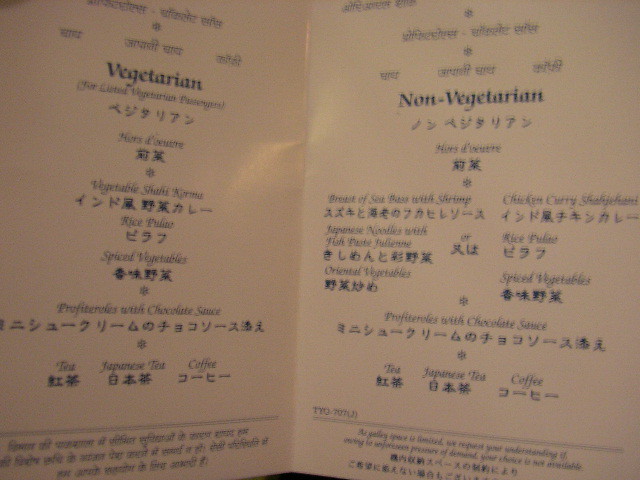This out-of-focus photo depicts a bilingual menu with a dark blue font set against a white background. The menu is two-sided, folding at a crease down the middle. The left side clearly labels a "Vegetarian" section, while the right side labels a "Non-Vegetarian" section. The text alternates between English and an Asian language, possibly Chinese, with English translations accompanying the Asian characters. Notably, "hors d'oeuvres" is presented in English with Asian characters below it. Both sides of the menu feature fine print at the bottom, though it is unreadable due to the poor focus. Decorative designs resembling either flowers or snowflakes divide the sections throughout the menu.